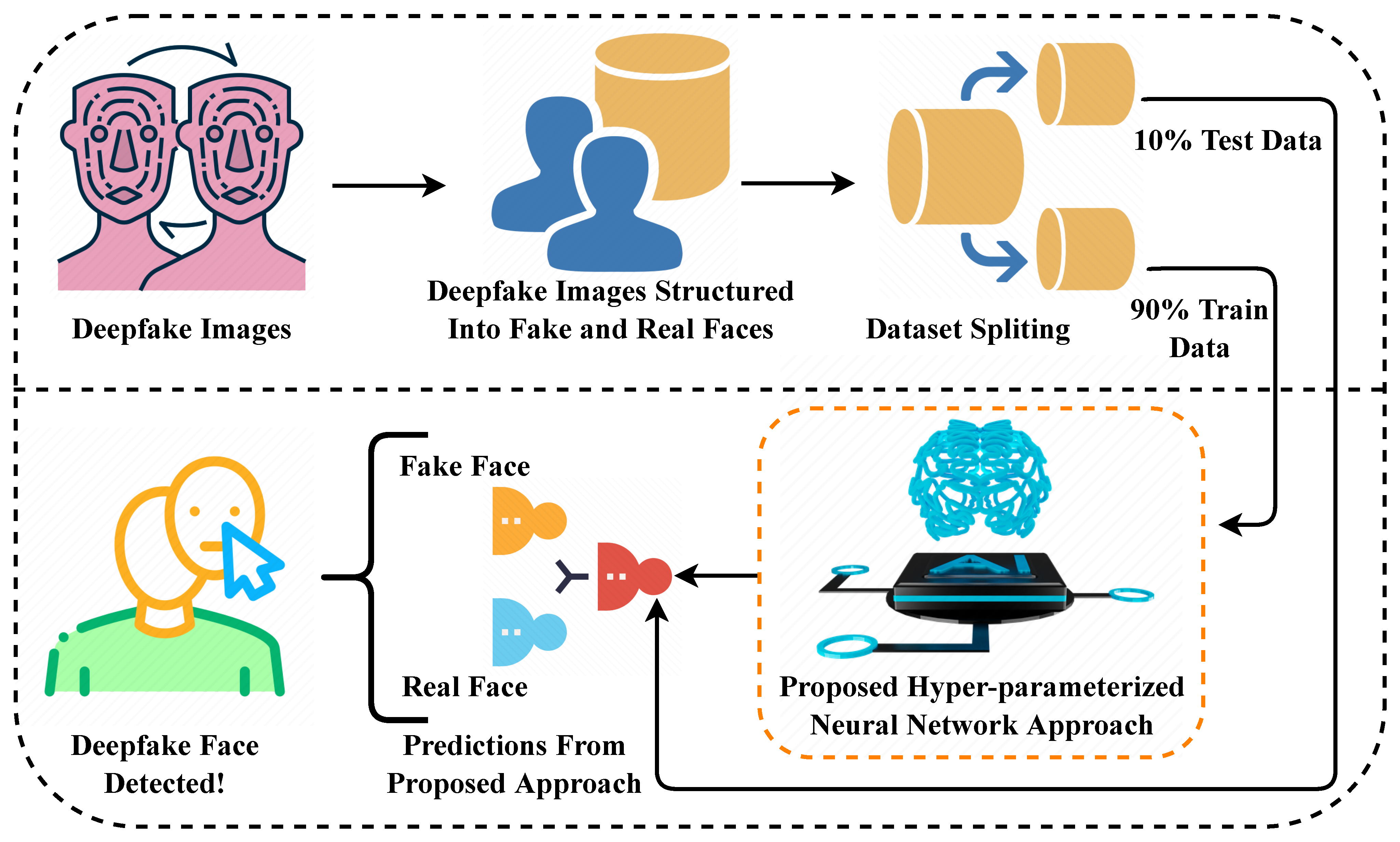The image is a detailed cartoon illustrated graphic in a rectangular format with a dashed outline, oriented with the longest side horizontally. The space is divided into two sections, with the bottom half slightly larger than the top. The illustration functions as an informative flowchart centered on the mechanics and identification of deepfake imagery.

At the starting point, there are two pink cartoon heads that represent the initial deepfake images. Arrows guide the flow from these pink heads to a stage where deepfake images are categorized into fake and real faces, depicted by two blue heads and a small circle nearby. The next stage involves a breakdown of the data used for deepfake structuring, with annotations highlighting that 10% is test data and 90% is training data. This is visually represented with a tube splitting into two smaller tubes, labeled 'data splitting.'

Following this, the flowchart presents an approach using a "proposed hyperparameterized neural network", illustrated with a black table and a blue drawing above it. Further arrows indicate predictions of 'fake face' or 'real face' generated from this neural network approach, accompanied by images of three colorful heads. The final segment of the flowchart points to a cartoon representation of a person's torso and face, featuring neutral facial expressions, with the label "deepfake face detected" signaling the outcome of the deepfake detection process.